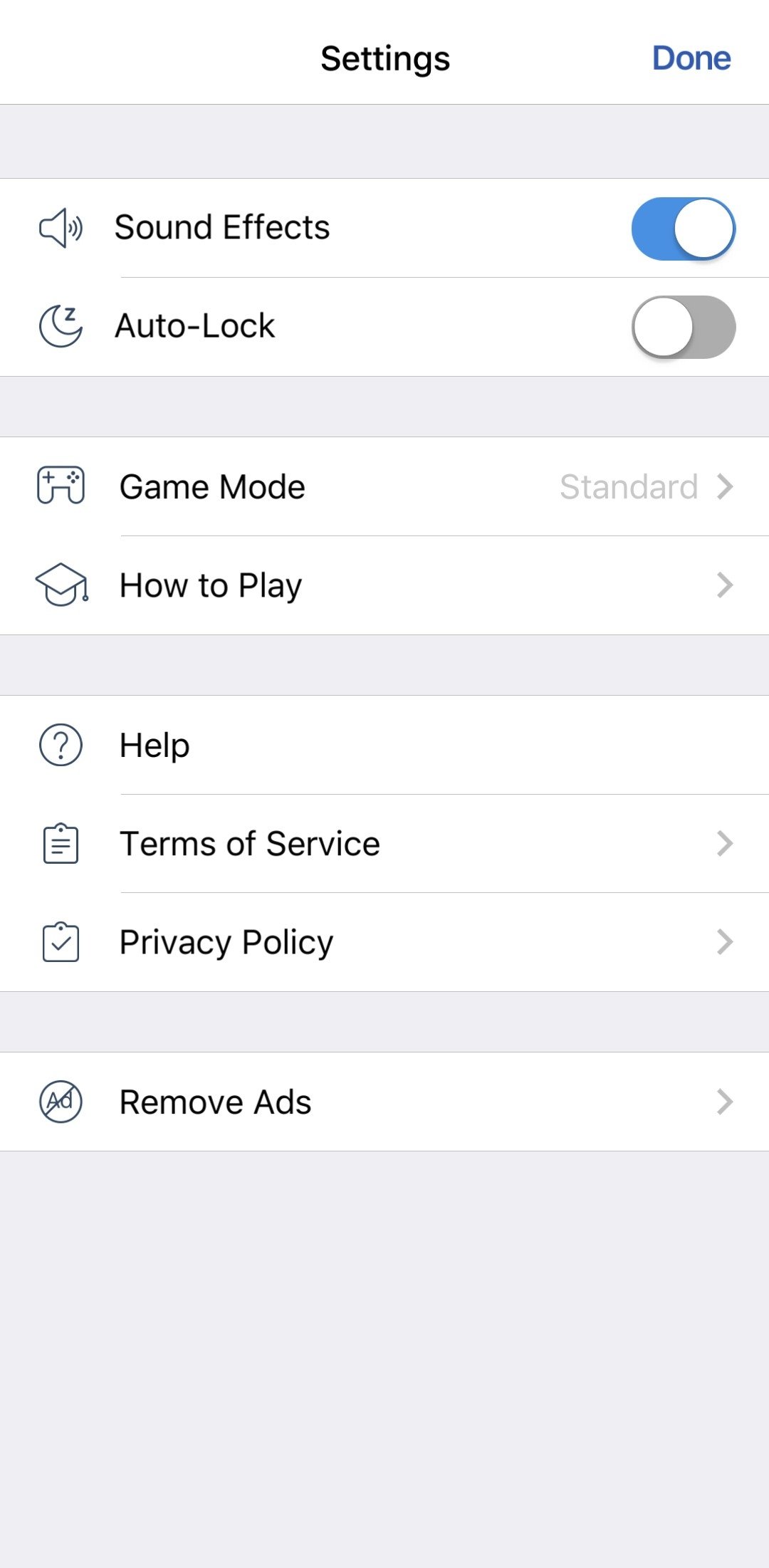Screenshot of a cell phone settings page. At the top, centered in bold black text, is the title "Settings," and on the right in blue text is the word "Done." Below this are the following elements:

1. A light gray rectangular header.
2. Two rows divided by a thin gray line:
    - First row: "Sound Effects" on the left with an icon beside it, and a blue toggle switch on the right indicating it is turned on.
    - Second row: "Auto-Lock" on the left with an icon beside it, and a toggle switch on the right that is turned off.

3. Another light gray rectangular header.
4. Three options with icons beside them:
    - "Game Mode" on the left with "Standard" in gray text on the right and a right-pointing arrow (sideways V).
    - "How to Play" on the left with a right-pointing arrow (sideways V) on the right.

5. Another light gray rectangular header.
6. Three options:
    - "Help" on the left.
    - "Terms of Service" on the left with a right-pointing arrow (sideways V) on the right.
    - "Privacy Policy" on the left with a right-pointing arrow (sideways V) on the right.

7. Another light gray rectangular header.
8. "Remove Ads" on the left with a right-pointing arrow (sideways V) on the right.

At the bottom of the screen is a large light gray rectangular footer that occupies the remaining space.